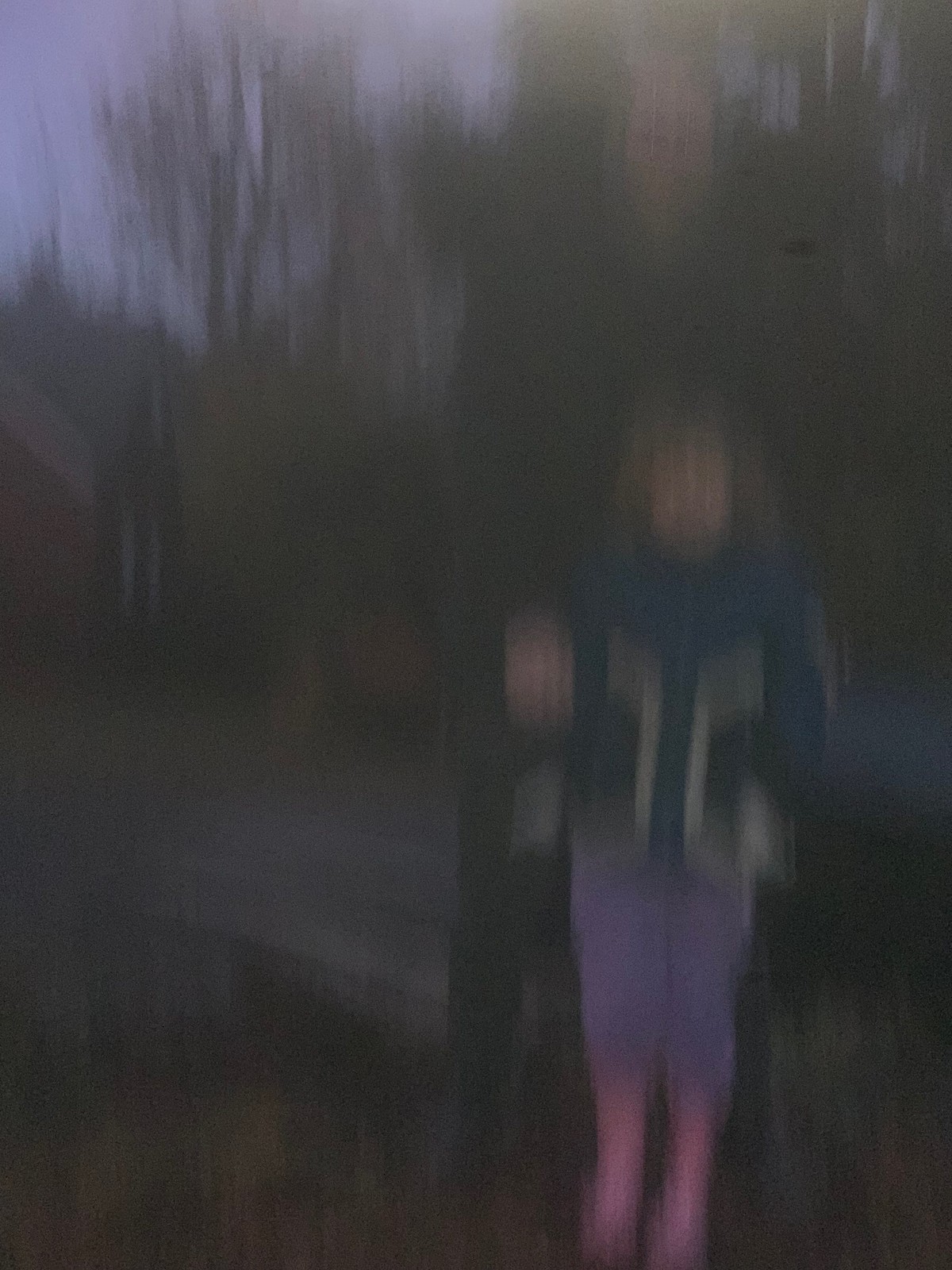A blurry, out-of-focus image depicts a white woman and a young girl standing together, seemingly caught mid-movement. The woman, with light brown and blonde hair, is dressed in dark-colored boots, pants, and a coat, her face obscured due to the camera motion. Her arm rests affectionately on the shoulder of the girl, who appears to be about six or seven years old. The girl has brown, slightly curly hair and wears a blue coat with beige detailing, purple pants, and pink rain boots. They are likely standing at the side of a road, as hinted by the presence of houses, trees, and a light blue sky in the background, indicating an outdoor setting.